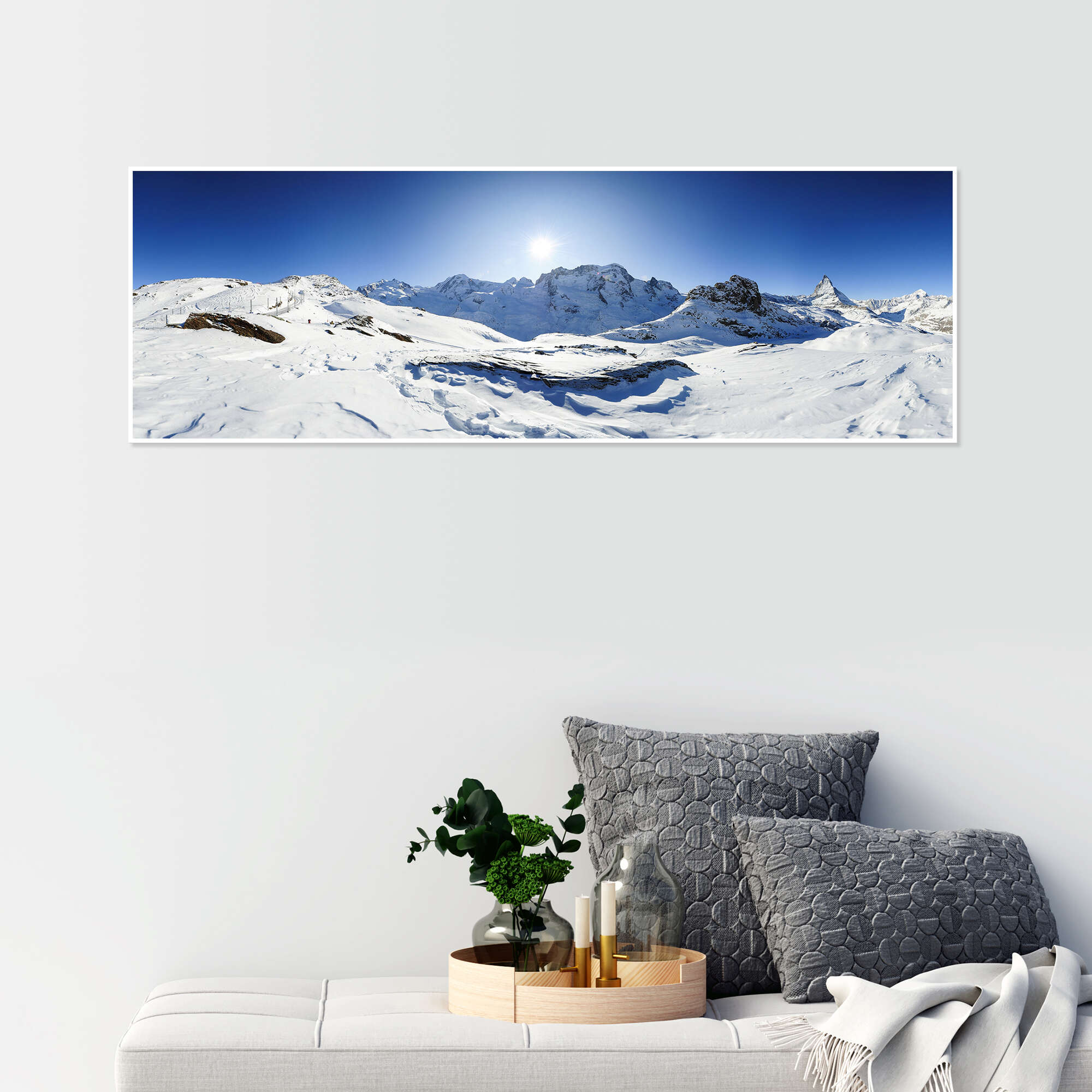The image features a serene room with a stark white wall, adorned by a stunning panoramic photograph of a snow-covered mountain range. The sun beams majestically from behind the mountains, casting a warm glow over the bright blue sky. Below the photograph, a small gray bench, soft-cushioned in white fabric, serves as a functional centerpiece. On the bench, there is a tan wooden organizer tray containing a variety of decorative items: a lush green eucalyptus plant in a vase, an empty glass bottle, and two stemmed candles in white holders with gold bases. Accompanying these are two textured gray pillows, one square and one rectangular, complemented by a white shawl draped casually over the bench. The overall composition combines elements of nature and coziness, creating a peaceful and inviting atmosphere.